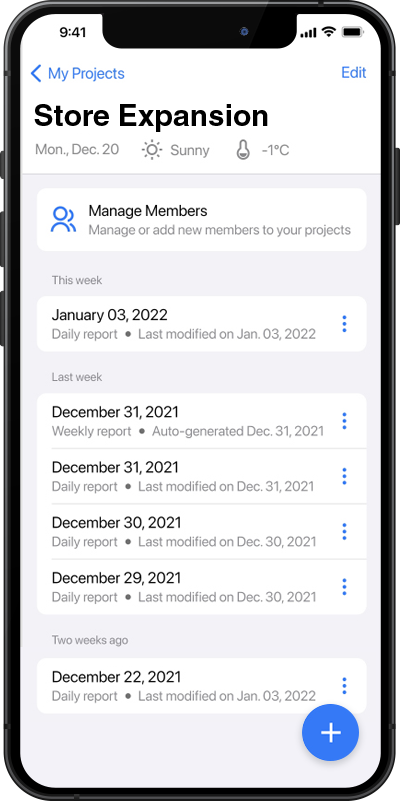The image depicts a smartphone displaying a collection of notes related to a project titled "Store Expansion." Each note corresponds to detailed daily entries, tracking activities from the last days of December 2021 through the first day of January 2022. The first entry begins on Monday, December 20th, noting "Sunny and -1°C" with a focus on managing team members, likely indicating efforts to add personnel to the project.

Highlighted entries include:

- December 22nd: The note indicates changes last made on January 3rd, 2022.
- December 29th: Mentioned as being modified on December 30th.
- December 30th: Another recorded entry.
- December 31st: Two separate notes are listed.
- January 3rd, 2022: The latest entry, modified on the same day.

The phone's interface shows a strong signal, with the time displayed as 9:41. The exact model of the phone is not specified, though it resembles either an Android or an earlier version of an iPhone based on its appearance.